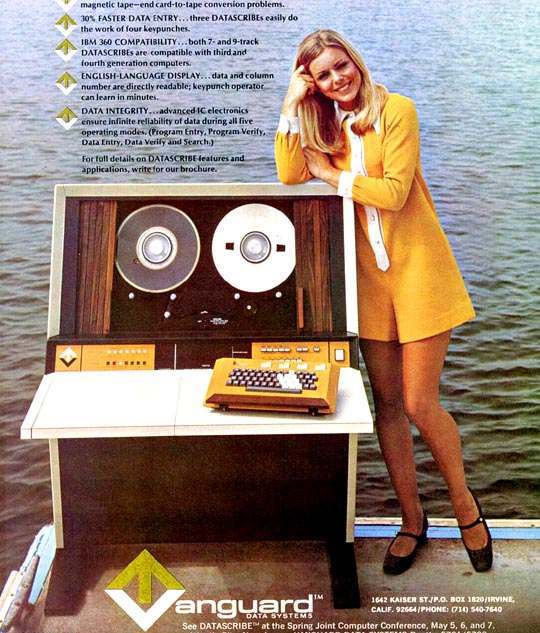This colorful scan of a vintage advertisement, likely sourced from an old magazine, features a striking image of a blonde-haired woman standing on a pier overlooking the ocean. She is dressed in a bright yellow romper with blue and white highlights along the sleeves and center buttons, complemented by black high-heeled shoes and a white necklace that drapes down to her waist. The woman is seen leaning on an old-style computer console, possibly from the 1960s or early 1970s, which showcases a wooden finish and is equipped with a yellow keyboard. The console features two large, spinning discs in its center and resembles a desk with a typewriter and a sound system. Above the computer, a bulleted list highlights key features such as "30% faster data entry," "IBM 360 compatibility," and "data integrity." The advertisement promotes Vanguard Data Systems, as noted by the text at the bottom of the image along with an address in Irvine, California.